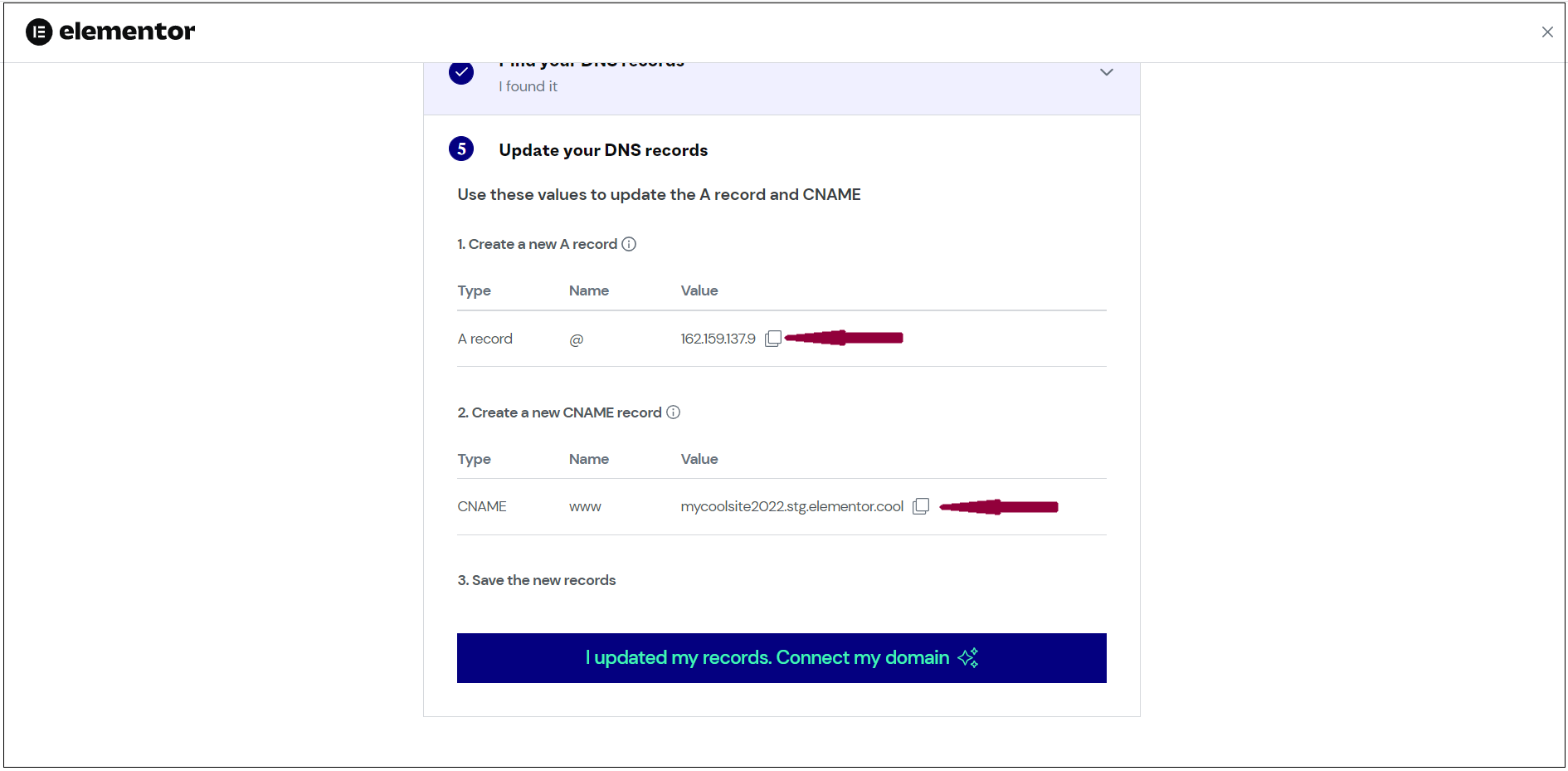The image features a user interface for updating DNS records on a website. The interface is centered, surrounded by large white margins on either side, giving it a minimalist look. At the top left corner of the interface, there is a black circular logo containing a stylized lowercase 'E,' next to which the word "Elementor" is written in lowercase black letters.

Beneath this branding, the main content of the user interface begins with the heading "Update your DNS records." The instructions are provided in a straightforward, text-heavy format. The steps are as follows:

1. Use these values to update the A record and CNAME.
2. Create a new record type: Name and Value.
3. Create a new CNAME record: Type, Name, and Value.
4. Save the new records.

Below these instructions, there's a prominent blue box containing a button with slightly seafoam green text that reads, "I updated my records, connect my domain." This button is likely the final step to confirm the updates made to the DNS records.

Overall, the image portrays an instructional web interface designed to guide users through the process of updating their DNS records, with clear branding and a user-friendly layout.